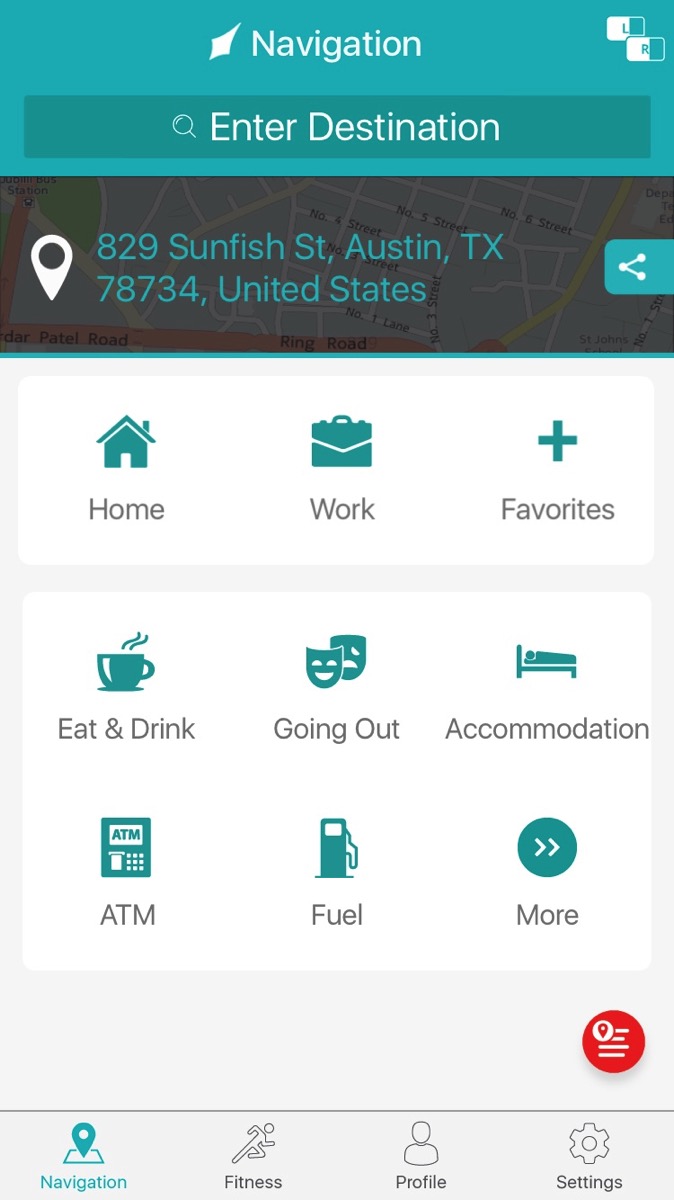**Detailed Caption:**

The image is a detailed screenshot of a navigation app. At the upper center of the screen, there is a prominent white navigation symbol accompanied by the word "Navigation" in white font. In the upper right corner, two squares contain the letters "L" and "R."

Just below the navigation title is a search bar with the placeholder text "Enter destination" in white font. Directly underneath the search bar, there's a location symbol which resembles a pin. Adjacent to this pin, an address is displayed in blue font: "829 Sunfish Street, Austin, Texas 78734, United States." To the right of this address, there's a turquoise-colored tab featuring a white share symbol.

Following this section, several menu icons are organized in rows. The first row includes icons labeled "Home," "Work," and "Favorites." Beneath them, the second row features "Eat & Drink," "Going Out," and "Accommodation." The third row consists of "ATM," "Fuel," and "More."

Towards the bottom right corner of the screen is a red and white symbol. At the very bottom, a row of navigation items includes icons for different functionalities: "Navigation," "Fitness," "Profile," and "Settings."